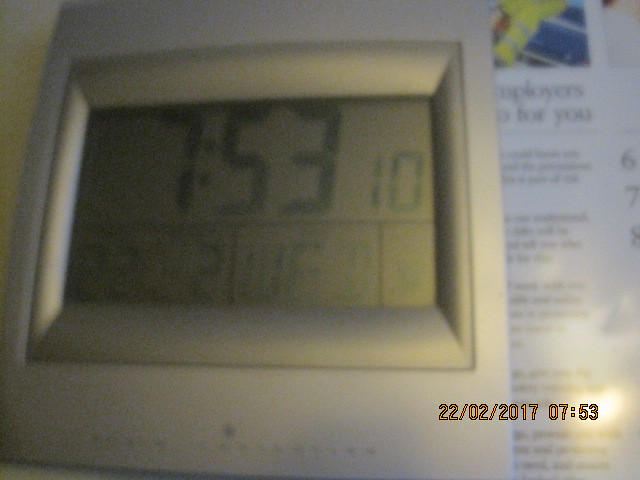The image presents a close-up, slightly blurry photograph of a gray, metallic-colored digital clock displaying the time "7:53" in large black numbers. Adjacent to the time, smaller text reads "10" seconds. The clock is framed by a slightly darker gray border on the digital display. Additionally, the clock features an orange timestamp reading "22-02-2017 at 7:53,” indicating the date as February 22, 2017. The lower right corner of the display includes another piece of digitized information, possibly the day, appearing as "T-U-E," suggesting it is a Tuesday. In the background of the image, there is a partially visible magazine or pamphlet with the words "employers" and "for you" discernible amidst the blur.